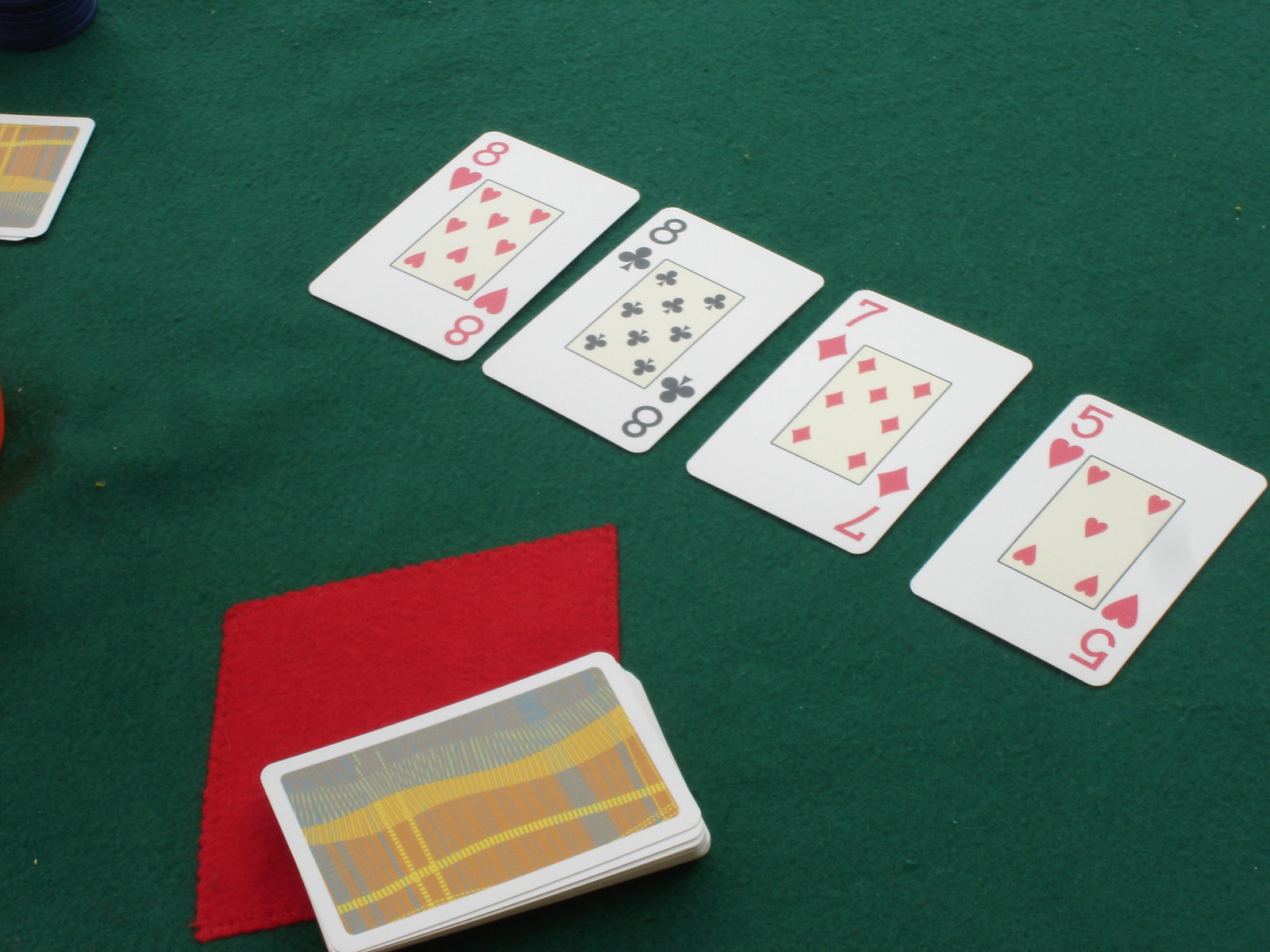The image features four face-up playing cards arranged in a line. From left to right, the cards displayed are: the five of hearts, the seven of diamonds, the eight of clubs, and the eight of hearts. The five of hearts and the seven of diamonds are both red cards, while the eight of clubs is black and the eight of hearts is red. 

At the bottom of the image, there is a stack of face-down cards. The back design of these cards features a cross-hatched pattern in gray, yellow, orange, and light blue. This stack is placed upon a square piece of red fabric, possibly a napkin. 

In the bottom left corner, partially cut off by the edge of the image, there are a few more face-down cards. The entire setup is laid out on a green felt surface, which has a noticeable rumple near the center-left area, suggesting it has been pushed up slightly. 

There is a dark shadow cast over this part of the image, as well as another shadow near the upper left corner, adding depth and contrast to the scene.